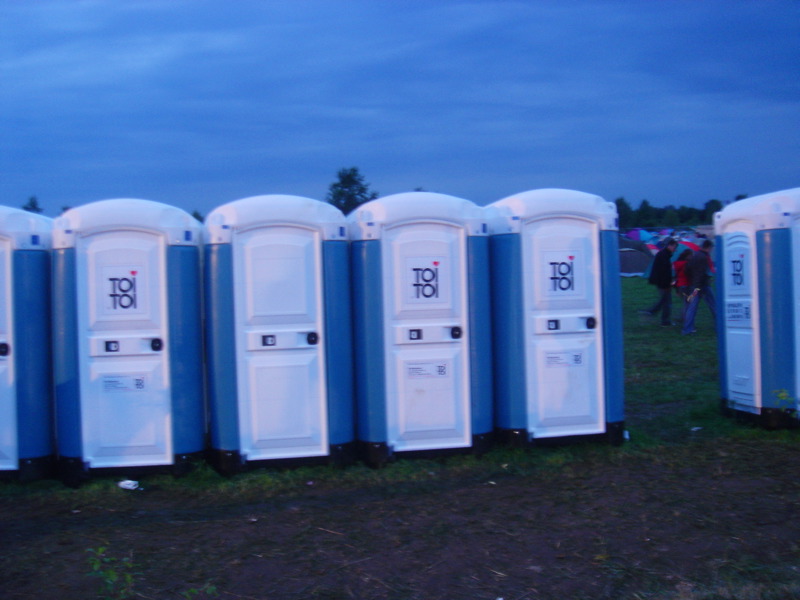This image is a color snapshot taken at dusk, capturing a festival or outdoor event. The evening sky is painted a periwinkle blue with traces of wispy white clouds, indicating that the sun is setting. Dominating the scene is a row of blue-and-white portable toilets, known as "Toy Toys," each adorned with a white roof, door, handle, and lock. Five of these portable restrooms are neatly lined up from the left center to the right, with a noticeable gap between the fifth and an additional one that is positioned separately and facing a different direction. The foreground consists of a muddy, dirty expanse with some grassy patches, creating a potentially sticky terrain. Behind the row of toilets, a line of green trees can be seen, and further in the distance, groups of people, bundled in coats, walk around, possibly heading back to their cars. There also appears to be some colorful parachute-like materials in the background, suggesting the possibility of a balloon festival. An apparent mix of black tarp or mulch lies in front of the portable toilets, contributing to the overall rugged and outdoor aesthetic of the scene.